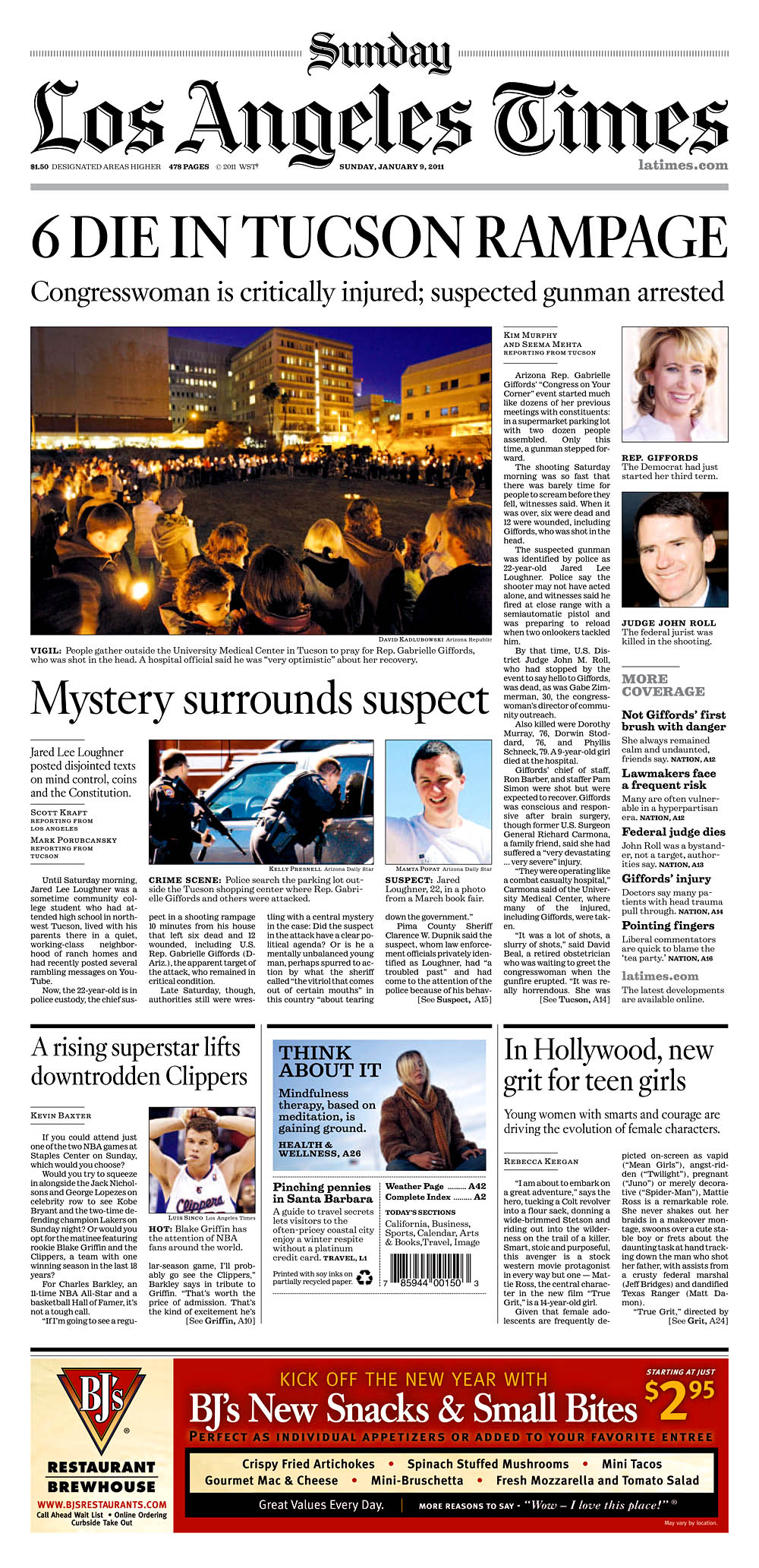A detailed caption for the described image:

"The front page of a Sunday Los Angeles newspaper features multiple articles and images. The main headline reads 'Tuscan Rampage: Congresswoman Critically Injured, Suspect Gunman Arrested,' accompanied by an image of people gathered downtown, holding lighters. Another article discusses the 'Mysteries Surrounding the Suspect,' illustrated with two photographs. A separate section highlights a story on a 'Rising Superstar Lifts Downtrodden Clippers,' and another article titled 'New Grit for Teen Girls in Hollywood' is also featured. Additionally, a promotion announcing 'BJ's New Snacks and Small Bites for $2.95' is prominently displayed with the price highlighted in yellow. The layout captures a mix of urgent news, human interest stories, and lifestyle updates."